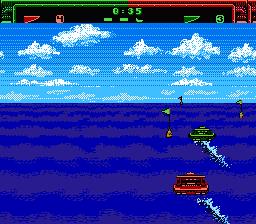This image captures a screenshot from a vintage 8-bit style video game, likely emulating the classic aesthetics of 1980s gaming. The scene depicts a boat race, with a dark blue ocean occupying the lower 55-60% of the frame. Two pixelated boats, one red and the other green, are positioned on the left, trailing light, foamy wakes behind them. Both boats share the same rectangular shape and feature distinctive exhaust pipes. They appear to be navigating towards three triangular buoys with green flags facing to the right.

Above the ocean, the sky is a vivid, animated blue with scattered white clouds, setting a lively backdrop for the race. Dominating the top of the image is a black banner displaying a green, 80s-style computer font countdown of "35 seconds" remaining in the game. This scoreboard section also features two sides: the green side has a red flag, and the red side has a green flag, marking each player's progress.

Overall, the image clearly evokes the nostalgic feel of early arcade or handheld video games with its pixelated graphics and simple, yet engaging, design.